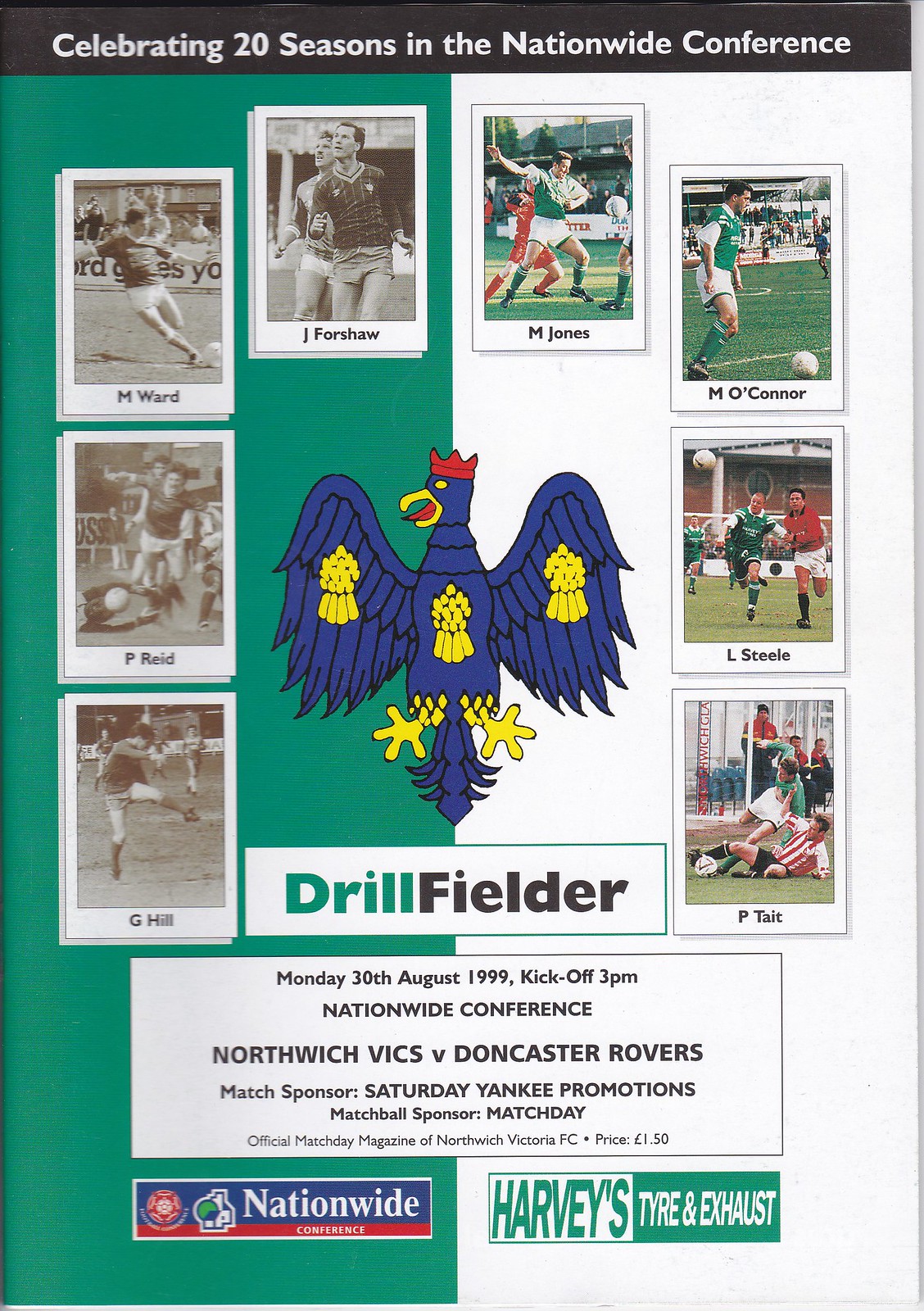The image is a scanned page from a magazine or program related to a soccer game, commemorating "20 Seasons in the Nationwide Conference." At the top of the page, there's a black bar with white text celebrating this milestone. Dominating the center of the page is a stylized, two-dimensional blue eagle with outstretched wings, featuring a red crown, a yellow beak, yellow eyes, yellow emblems on its wings, yellow feet, and a yellow chest. Below the eagle is the text "Drill Fielder" in green and black.

The layout of the page includes eight photographs of various soccer players. The left column, with a green background, includes black-and-white photos of J. Forshaw, M. Ward, P. Reid, and G. Hill from top to bottom. The right column, on a white background, features color images of M. Jones, M. O'Connor, L. Steele, and P. Tate from top to bottom. Additional images are positioned above the eagle.

A white rectangle beneath the eagle provides details about a specific match: "Monday, 30th August 1999, kickoff 3 p.m., Nationwide Conference. Northwich Vicks vs. Doncaster Rovers." It lists the match sponsor (Saturday Yankee Promotions), the matchball sponsor (Match Day), and mentions that it is the official matchday magazine of Northwich Victoria FC, priced at £1.50. Along the bottom are corporate logos for Nationwide and Harvey's Tire and Exhaust, with "tire" spelled "T-Y-R-E".